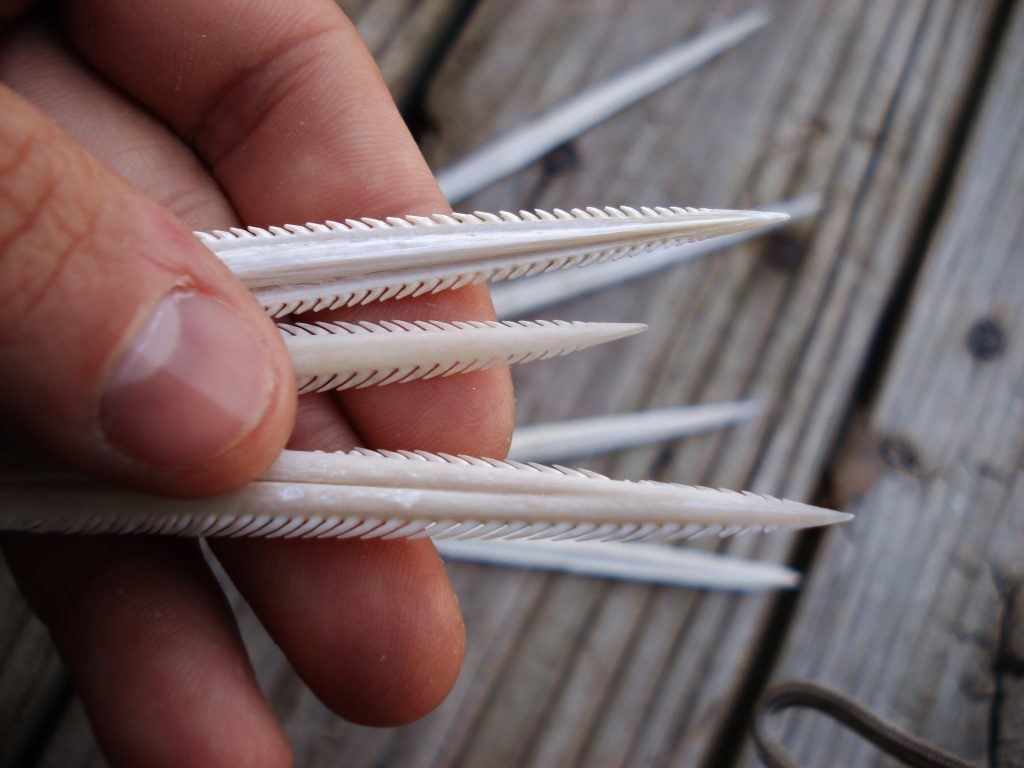In this close-up photo, a person's hand, entering from the upper left corner, is prominently featured holding three small, white, bone-like objects with ridges along their length. The thumb is positioned over these objects, securing them while the tips of the forefinger, middle finger, and ring finger support them from below. These objects are pointed at the ends and display a distinct pattern of ridges on either side. The bottom object is the most visible, with its ridge formations clearly seen, curving down and back at the top and up and back at the bottom. The second object partially peeks out from under the thumb, and the third extends slightly upwards, overlapping the forefinger.

In the background, several more of these bone-like objects are placed on worn wooden boards. These boards, displaying signs of wear and rust around their nails, suggest an outdoor setting. Additional elements, such as a hook, hint at a fishing or exploration context, possibly implying the objects could be fishing tackle or artifacts discovered during a journey. The overall scene captures the rustic and somewhat mysterious ambiance of the setting, providing a glimpse into an intriguing moment frozen in time.